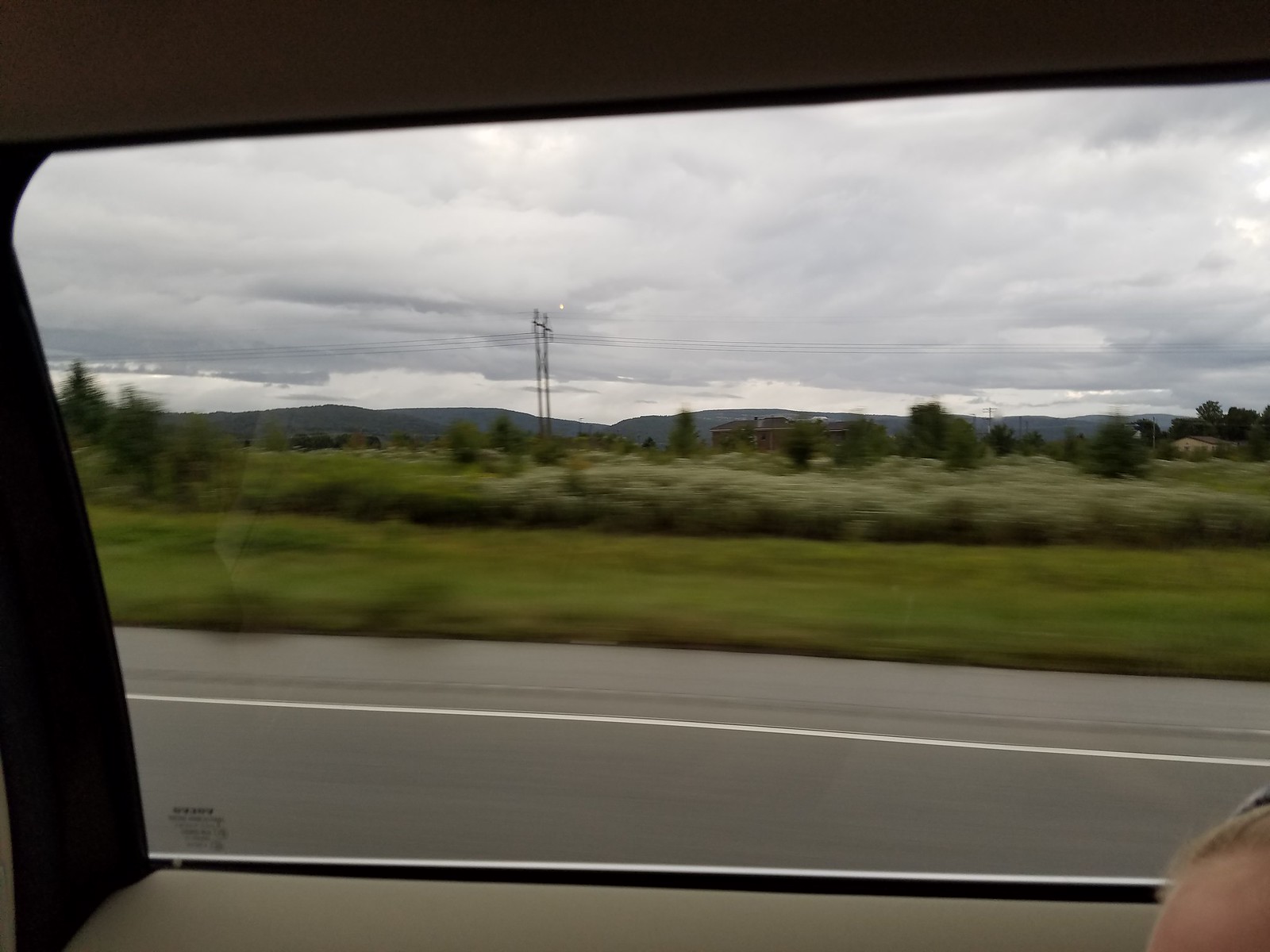A photograph captures a panoramic view from inside a car, looking out through the passenger window. Dominating the background are majestic mountains set against a somber, gray sky. Crisscrossing the scenery, high-tension electric wires add an industrial touch. In the foreground, abundant with long grasses and weeds, a partially obscured house peeks through dense trees. Another tan house with a brown roof is visible further back but is similarly shrouded by sparse trees. Between the wild growth and the highway lies a somewhat manicured lawn.

The highway itself, made of black asphalt, features a white line demarcating a bicycle lane. Inside the car, the tan interior is visible along with a small sticker on the window, likely indicating the brand. Intruding into the frame at the very bottom right corner is a portion of someone’s forehead with a hint of blonde hair, adding a human element to the scene.